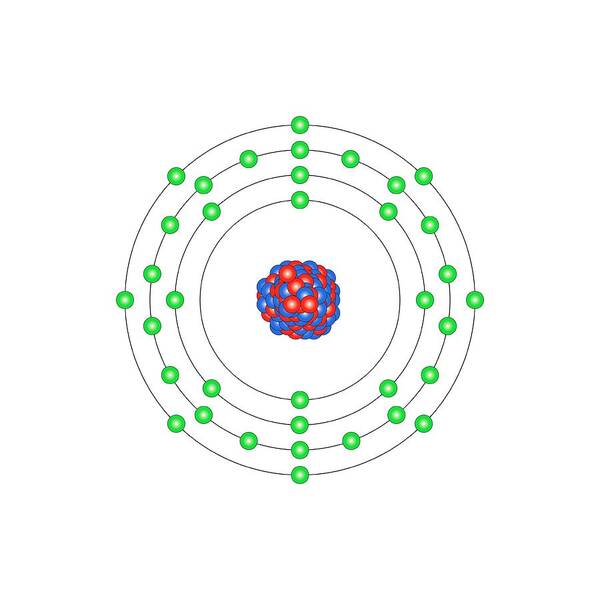The image portrays a digital line drawing of concentric circles, each adorned with multiple green dots, giving the appearance of cellular structures. There are precisely four outer circles encircling a central pattern composed of overlapping red and blue circles. The colors used in the drawing include black, white, green, red, and blue, with no additional background, creating a scientific and minimalist aesthetic. The graphic, reminiscent of atomic or cellular illustrations, could be suitably placed in a scientific site, textbook, or educational poster. Each outer circle features green dots that are consistently arranged vertically, while other dots follow a distinct yet organized pattern around the central motif. The meticulous arrangement and limited color palette suggest a focus on clarity and informational value.